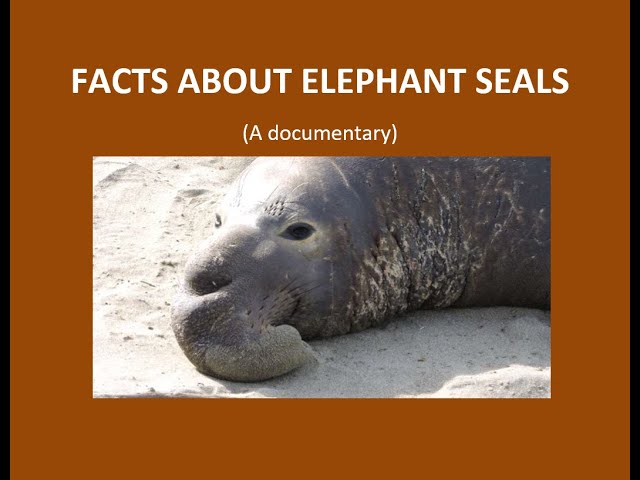The opening slide of a documentary presentation titled "Facts About Elephant Seals" features a simple yet evocative design. The backdrop is a burnished brown-tan, framed by black borders about a quarter-inch thick on the left and right sides. Centered in this frame is a compelling image of an elephant seal sprawled on a white sandy beach. The seal's face—complete with open eyes, a mouth dusted with sand, and notable skin markings—draws immediate attention. The white text above the image reads, "Facts About Elephant Seals: A Documentary," suggesting that this slide is part of a PowerPoint or Google Slides presentation. The overall design hints at a straightforward yet informative exploration of these fascinating marine mammals.